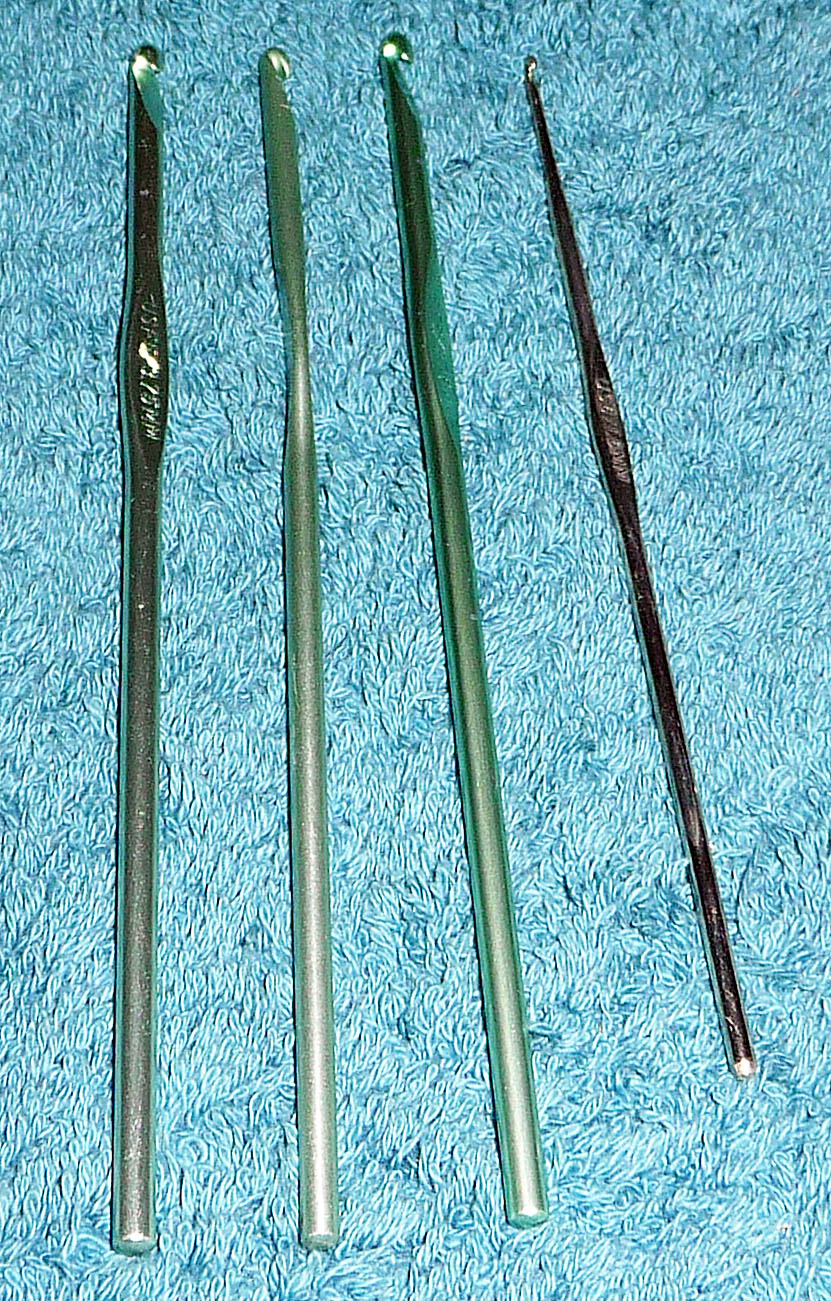This close-up color photograph captures four metal crochet needles laid out on a turquoise shag carpet. The needles, composed of shiny, silvery metal with slightly different shades, are arranged diagonally from top left to bottom right. The three larger needles, each with a cylindrical body that flattens towards the top, end in small curved hooks – features characteristic of crochet tools. The fourth needle on the far right is notably smaller and thinner, with its flattened section appearing much sooner along its length compared to the others. A light source from the bottom right gently illuminates the scene, making the metallic surfaces glisten. The needles, used and slightly worn, rest against the textured fibers of the carpet, which showcases a mix of light blue shades.